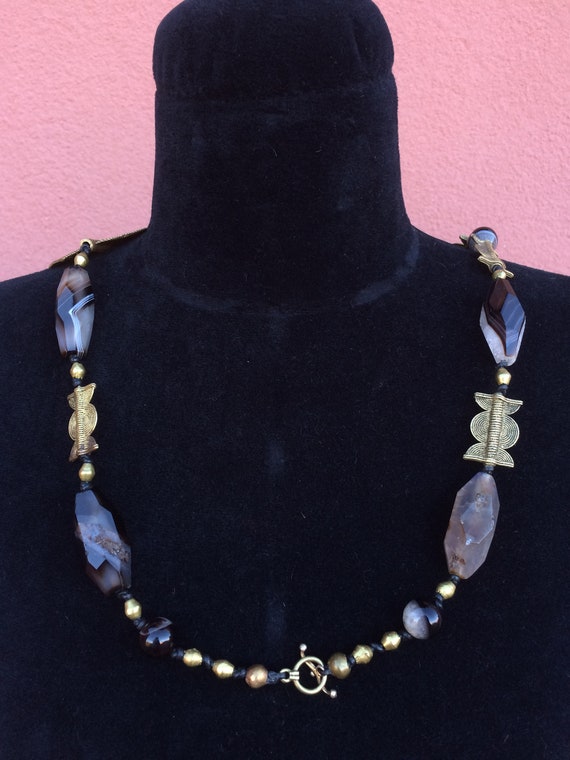This image captures a handcrafted necklace displayed on a black mannequin bust with a suede or felt lining, set against a pink or light fuchsia wall. The mannequin, representing the chest and neck without a head, highlights the intricate details of the necklace. The necklace is composed of various gemstone beads, including oval-shaped dark black and quartz-like stones, interspersed with small gold beads and connectors. The design features an artistic arrangement of elongated and round gemstones, along with flattened metal pieces, such as a circular shape bordered by two half circles. At the very bottom, a golden clasp is visible, adding a functional yet elegant touch to the overall piece. The ensemble creates an eye-catching, sophisticated look that draws attention to the meticulous craftsmanship and the harmonious blend of materials.